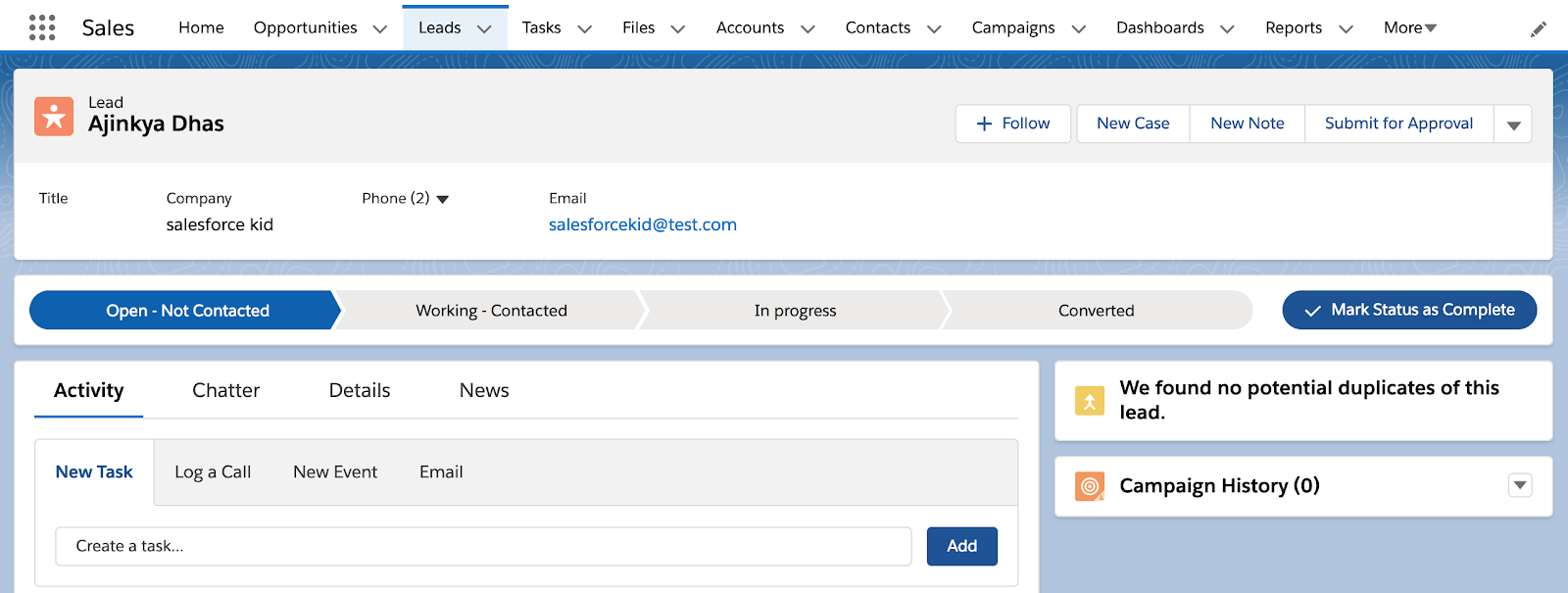Screenshot Description:

This screenshot showcases a comprehensive view of a webpage on a website. At the top, there is a horizontal navigation menu featuring several options neatly listed out for ease of access. On the leftmost side, there are nine dots arranged in a three-by-three grid, suggesting a menu or additional features. Adjacent to these dots, the word "Sales" is displayed, followed by the main navigation items: Home, Opportunities, Leads, Tasks, Files, Accounts, Contacts, Campaigns, Dashboards, Reports, and more. The "Leads" option is highlighted in blue, indicating the current selection on the page.

On the far right, there is a pencil icon at the top corner, offering options to edit or write a particular item. Beneath this, on the left-hand side, there’s an icon of a person encased in a star within an orange square. The label "Lead" is present alongside the name "Ajinkya Das." Further details include the title "Company: Salesforce Kid," a phone entry with a "2" in parentheses, and an email address highlighted in blue: "SalesforceKidAtTest.com."

Above this section, on the right, there are several actionable buttons: "Follow," "New Case," "New Note," "Submit for Approval," and a dropdown arrow for additional options. Directly underneath, a progress tracker displays the current status in the website: "Open, Not Contacted" is highlighted in blue, followed by stages such as "Working Contacted," "In Progress," and "Converted." To the right, there is an option to "Mark Status as Complete" in blue.

Towards the bottom, a set of navigation tabs are available: "Activity," "Chatter," "Details," and "News." The "Activity" tab is underlined in blue, indicating it's currently active. Within this tab, additional options like "New Task," "Log a Call," "New Event," and "Email" are provided, along with a search bar at the bottom for task creation.

On the right side of this section, two informational icons can be seen. The first icon of a person walking inside a yellow square states "We found no potential duplicates of this lead." Below it, another icon featuring a target within an orange square indicates "Campaign History" with a zero in parentheses.